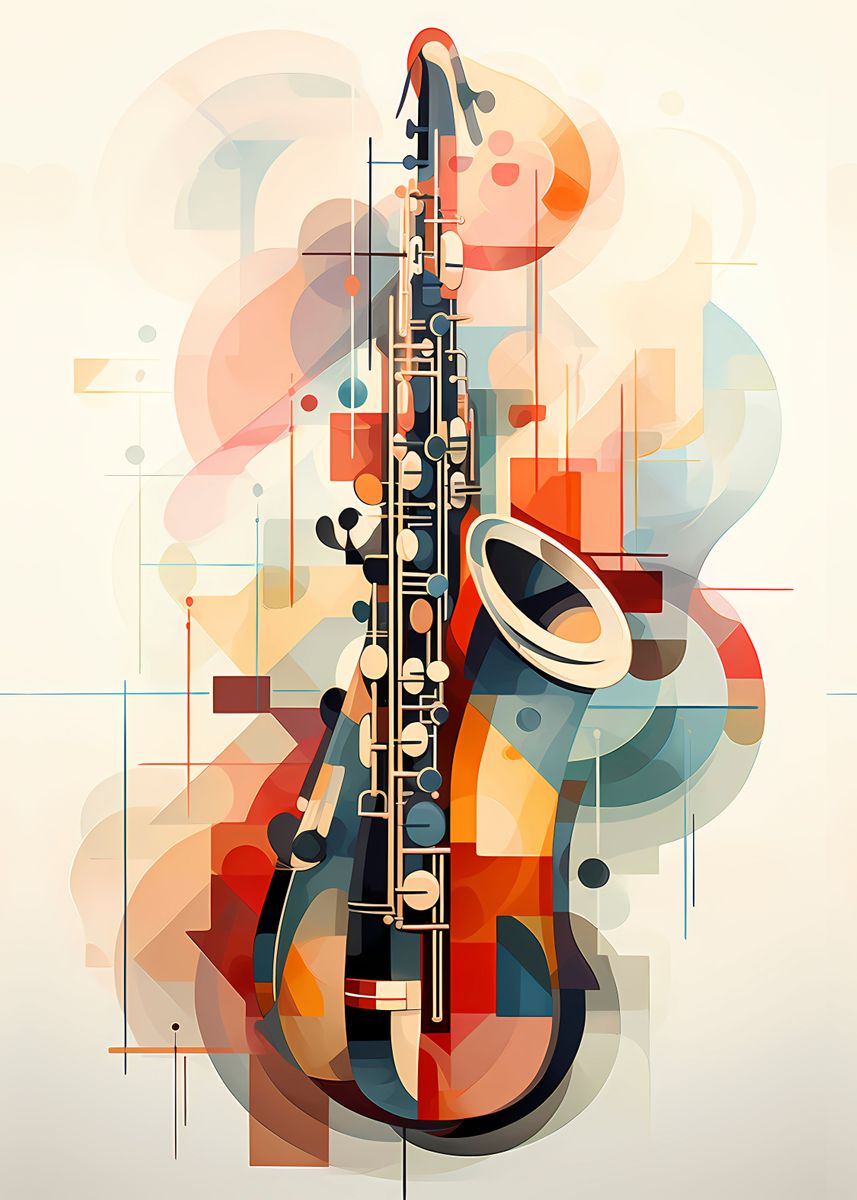This image is an abstract, computer-generated artwork depicting a saxophone created using a diverse palette of geometric shapes and vibrant colors. The saxophone itself is composed of an intricate array of blues, oranges, reds, yellows, and pinks, forming a striking contrast against a light pinkish-peach background. The saxophone's valves and mouthpiece are rendered in a mix of these colors, with some of the key circles represented in tan, blue, and orange. The background complements the main subject with an assortment of colorful straight lines, dots, and circles, alongside red squares, boxes, and triangles, maintaining a cohesive geometric and abstract theme. The overall artwork exudes a pastel quality, blending lines, blobs, and shapes to create a visually engaging representation of the saxophone, making it a vibrant piece suitable for wall display.